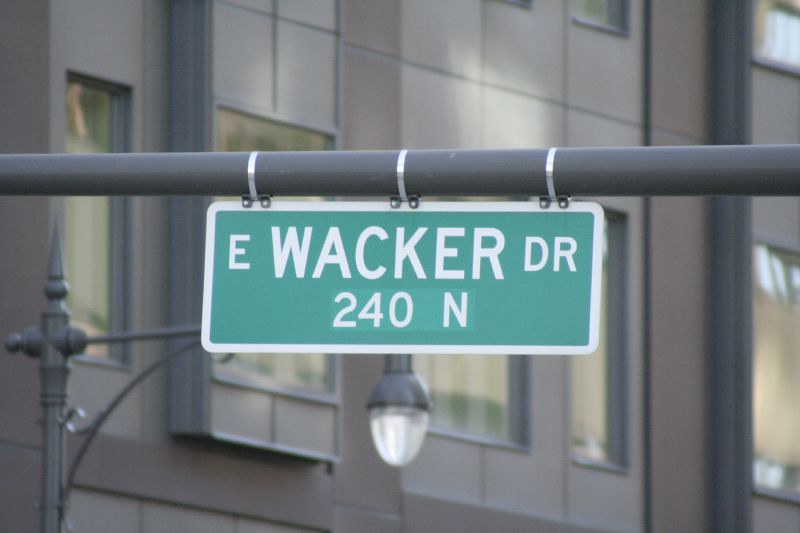This close-up photograph showcases a horizontally mounted green street sign, firmly attached to a pole with three visible ties. The pole extends from the upper left to the upper right of the frame, positioning the sign prominently in the center. The sign itself is elongated and thin, featuring a bold green background with a white border. In distinct white lettering, the larger word "Wacker" is centered, flanked by a smaller "E" on the left and a smaller "DR" on the right. Below these inscriptions, the designation "240 N" is clearly visible.